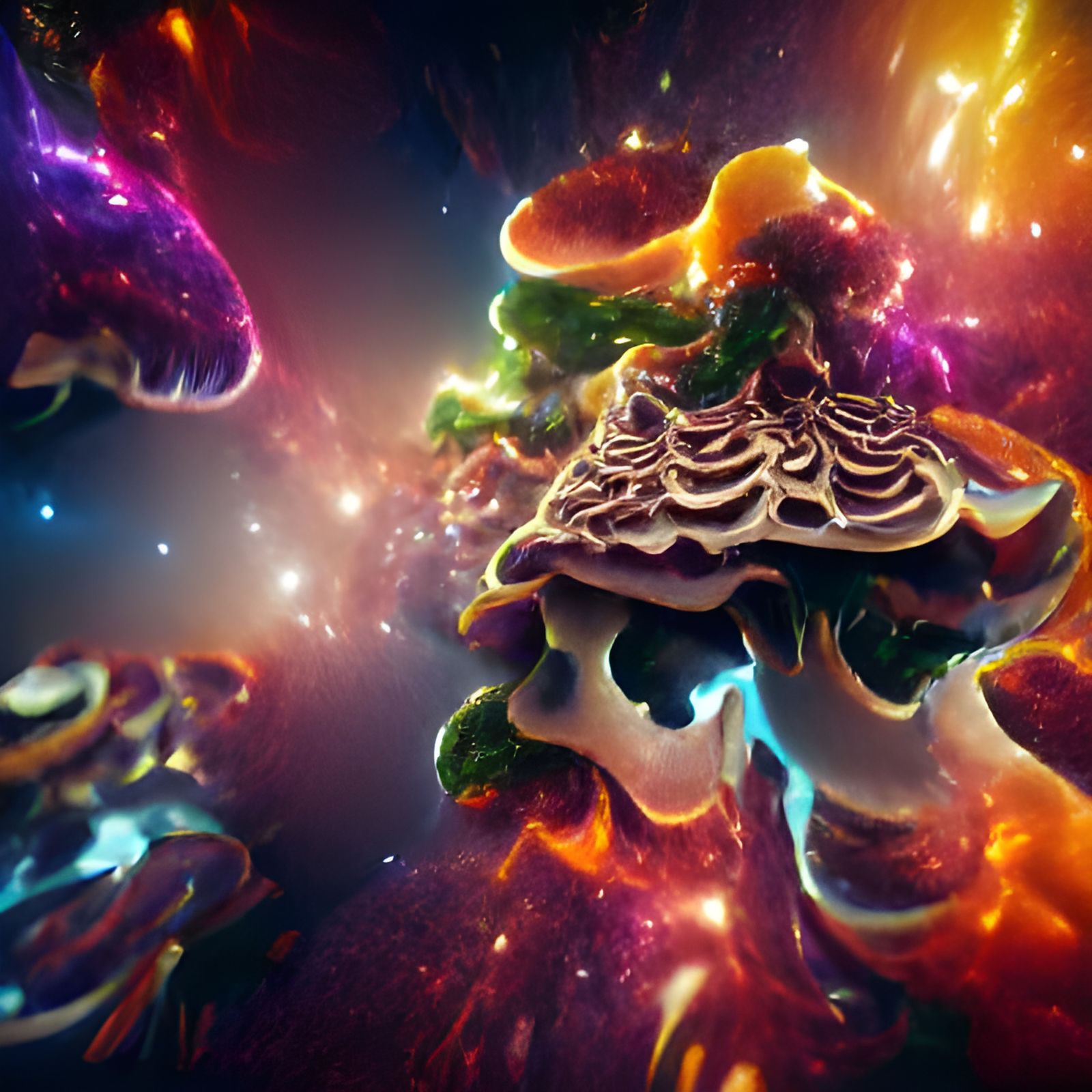This digital image is a mesmerizing, highly detailed piece of conceptual or abstract art that blends elements of psychedelic and outer space themes. In a square format, it radiates with vibrant, almost neon glows across its various hues. The right side of the image is dominated by bright oranges, reds, and pinks, mingling with whites and greens around mushroom-like shapes. The center features dark, black areas punctuated with bright, glowing spots, creating a stark contrast. On the left, blues and purples form undulating shapes that resemble coral or a whale's face seen in a trippy vision. The lower sections have detailed renditions of mushroom-like forms with colorful bases, including an eye-catching white mushroom accented with greens, purples, and oranges. This piece has an impressionistic quality, evoking both a sense of flowing lava and the serene depths of the ocean with its dreamy, psychedelic patterns, indicating it might be a 3D rendering. The overall effect is both dark in background but bursting with rich, shiny, and vibrant colors, capturing the viewer's imagination with its surreal, otherworldly scene.